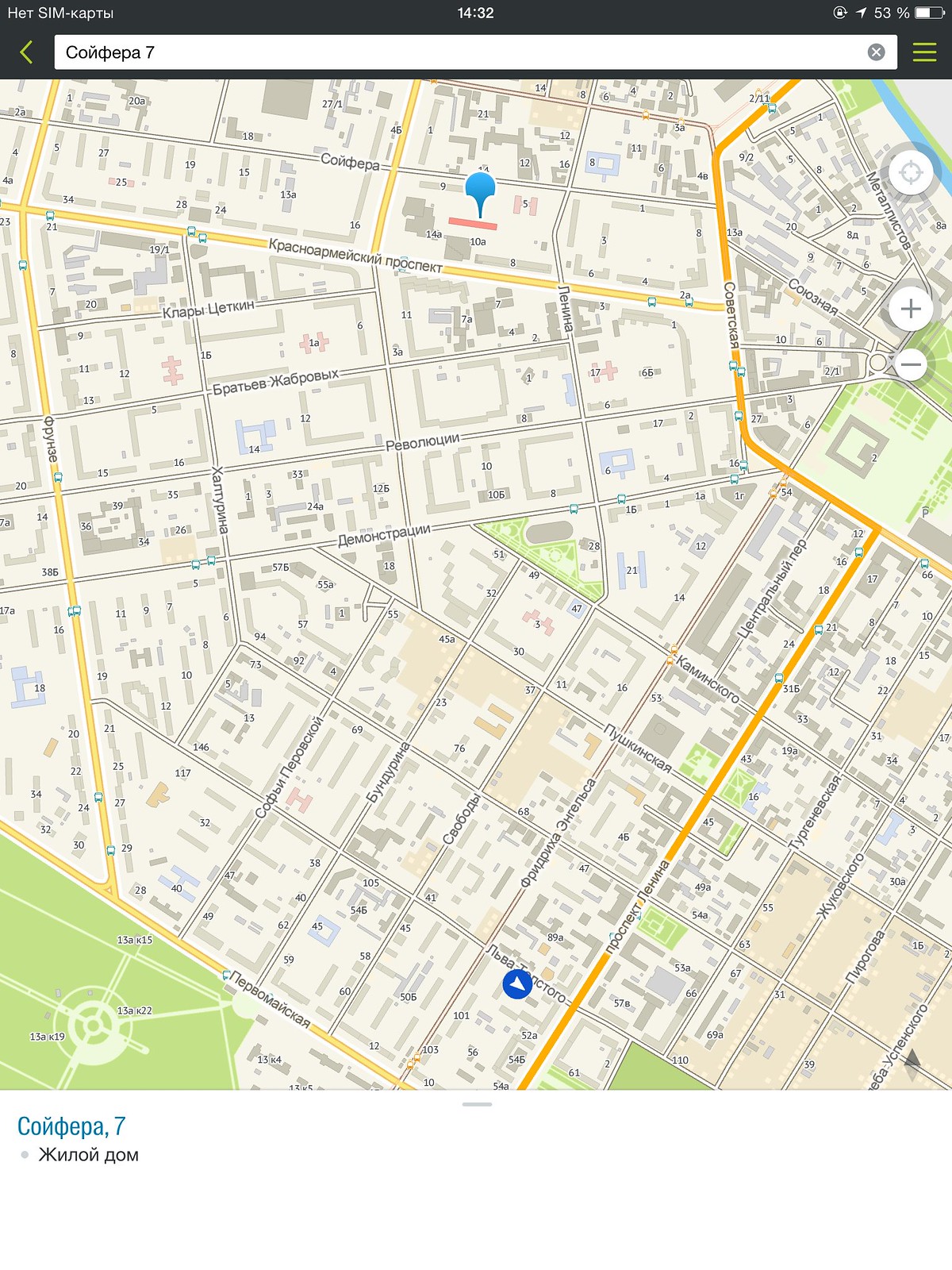This photograph captures a screenshot of a map displayed on a cell phone. At the top of the image, the label "hot sim" is followed by the letters "k-a-p-t-w," suggesting the use of a different language, possibly Russian. The time, displayed prominently in white text at the center-top of the screen, reads 14:32, while the battery level on the right side shows 53%.

Examining the map itself, we observe a variety of road colors: yellow roads dominate the left side, extending towards the right, interspersed with mostly white roads that likely represent side streets. On the right side of the map, an orange road descends towards the middle, hinting at its importance as a main thoroughfare. Notably, a blue circle with a white arrow represents the user's current location, positioned near the bottom-middle of the map. This circle assists in pinpointing the specific area the user is navigating.